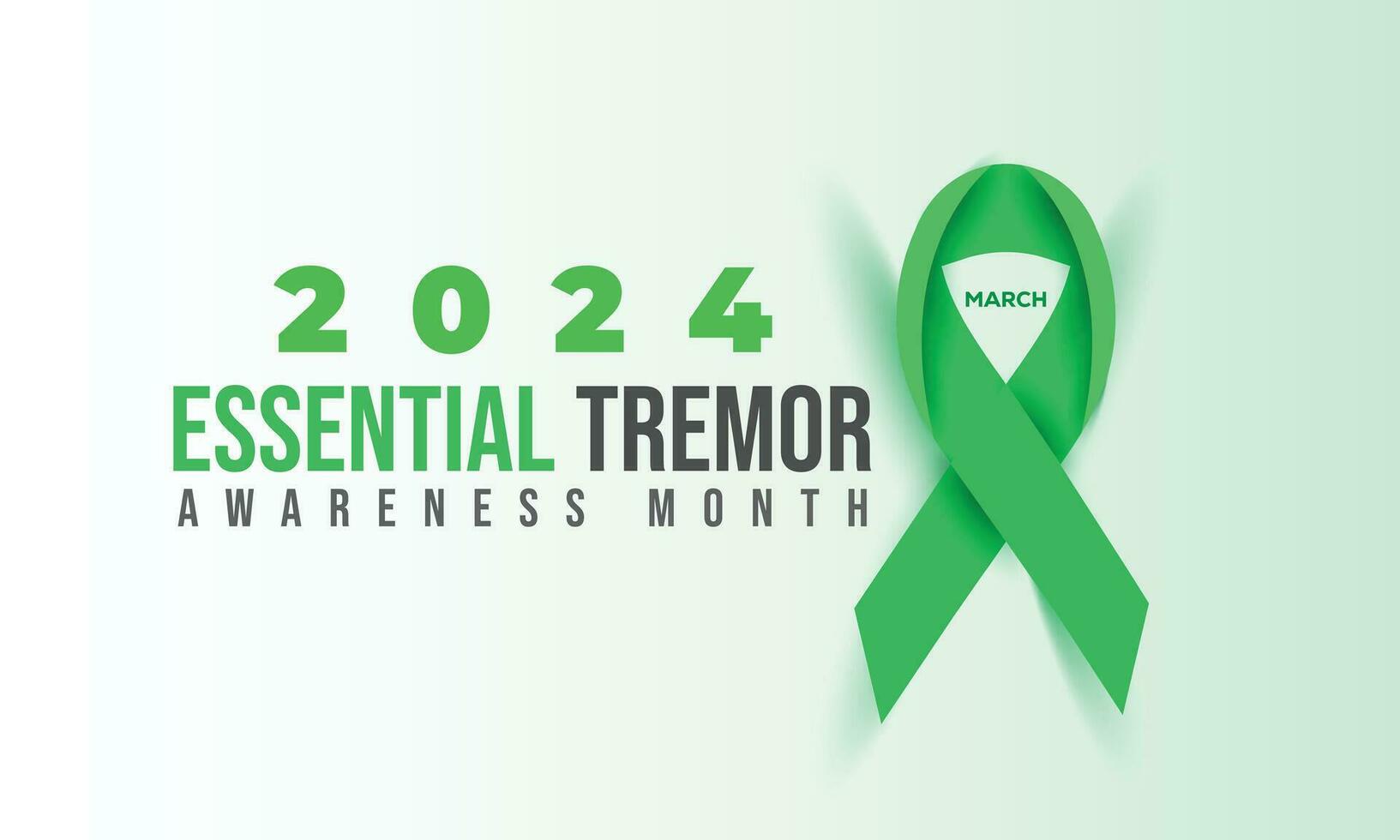This image is a detailed advertisement for the 2024 Essential Tremor Awareness Month. It features bold, wide block letters spelling out "2024 Essential" in green. Below that, "Tremor" appears in purple, followed by "Awareness Month" in a dark blue or black font. The background transitions from white on the left to a light mint green towards the right, creating a gradient effect. On the right-hand side of the image, there is a prominent green support ribbon with a loop at the top and crossed ends. The ribbon casts a light shadow and has the word "March" printed in its center. The design is visually striking yet simple, aiming to raise awareness with clarity.